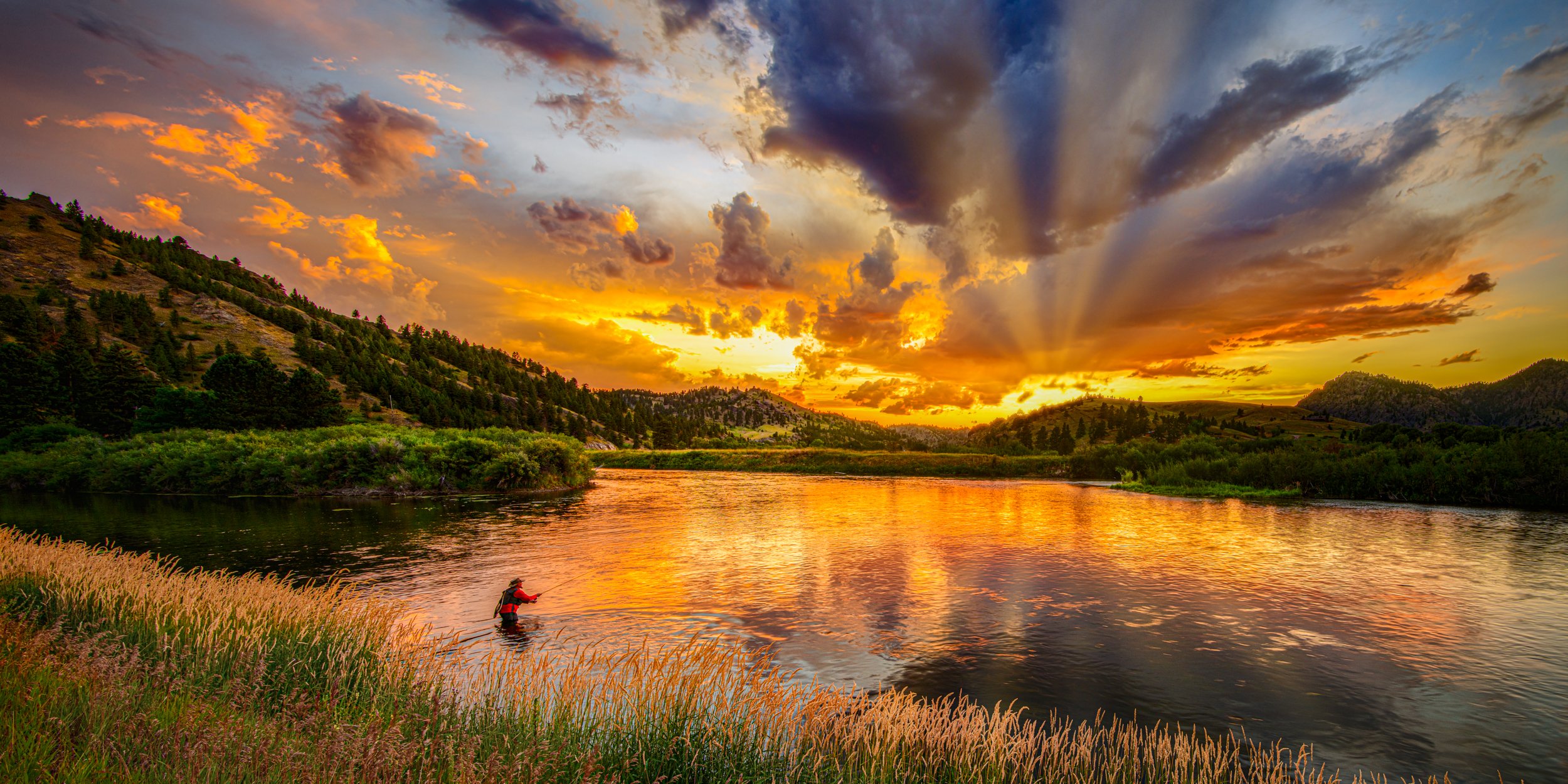In this stunning photo of a serene, outdoor landscape, a large body of water dominates the bottom portion, showcasing two lake streams merging effortlessly. A gentleman, clad in a red long-sleeve shirt and thigh-deep in water, is engaged in fly-fishing near the bottom left corner. His fishing pole is barely discernible, catching the eye with its delicate arc. This vantage point from a grassy hill reveals tall grasses along the edge of the calm river, where low bushes and trees are sporadically placed along the banks.

The horizon is adorned with a breathtaking sunset, featuring a palette of golden yellows, bright oranges, purples, and blues that casts a vibrant reflection on the water's surface. Rays of light pierce through scattered dark clouds, adding a dramatic contrast to the clear sky. The background is graced with mountains that stretch across the scene, some of which are tree-covered. The sun majestically sets behind these mountains, creating a peaceful and radiant ambiance with its colorful display, mirrored vividly in the tranquil water below.